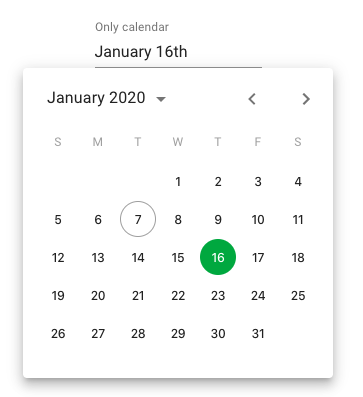The image is a screen capture from an application or website displaying a calendar interface. At the very top, on a simple white background, it reads "Calendar, January 16th." Below, a rectangular calendar is set against a subtly different white background, accentuated with a drop shadow for clear distinction.

The header of the calendar reads "January 2020," accompanied by a downward-facing arrow, indicating a dropdown menu for selecting different dates. To the right are left and right arrows, allowing navigation between months. Below the header, the days of the week are represented by single letters: "S M T W T F S." The calendar grid starts with "1" on a Wednesday and ends with "31" on a Friday. 

Specific dates are highlighted: Tuesday the 7th is encircled with a gray ring, while Thursday the 16th is marked by a filled green circle. These highlights likely denote events, appointments, or possibly holidays, although no common holidays fit these specific dates in January.